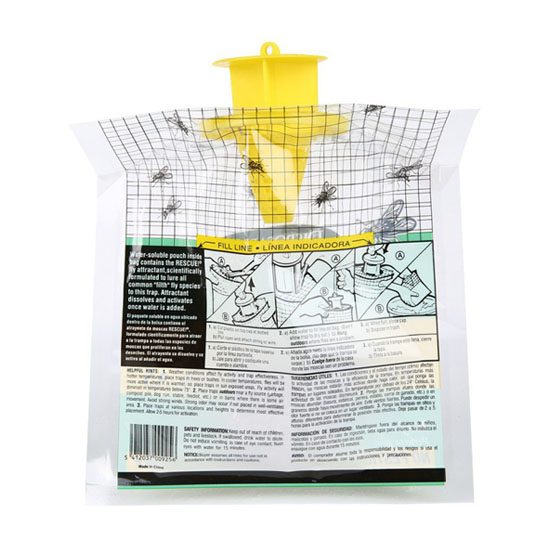This photograph showcases the back of a clear plastic fly-catching device or trap, prominently featuring a yellow plastic cap that fits into the top of the vertical rectangular bag. The cap itself has a triangular bottom and a cylindrical top. Surrounding the top 40% of the bag is a black-outlined grid pattern, adorned with illustrations of flies, giving the impression of a screen with flies on it. Directly beneath this, there’s a yellow bar labeled "fill line."

To the left side, there’s a large black box filled with white text, although the specific wording is unreadable due to the image quality. Adjacent to this black box to the right, there are three distinct panels featuring visual instructions on the device's usage. These panels illustrate how to pop open the yellow cap and add water or an attractant mixture, explaining the process by which flies enter the trap and get caught.

Further down, there is additional text in black, written against white backgrounds, which provide more detailed instructions or product information but are difficult to decipher clearly. A barcode is visible in the bottom left corner of the bag, along with a black bar at the very bottom, carrying more text that remains too small to read.